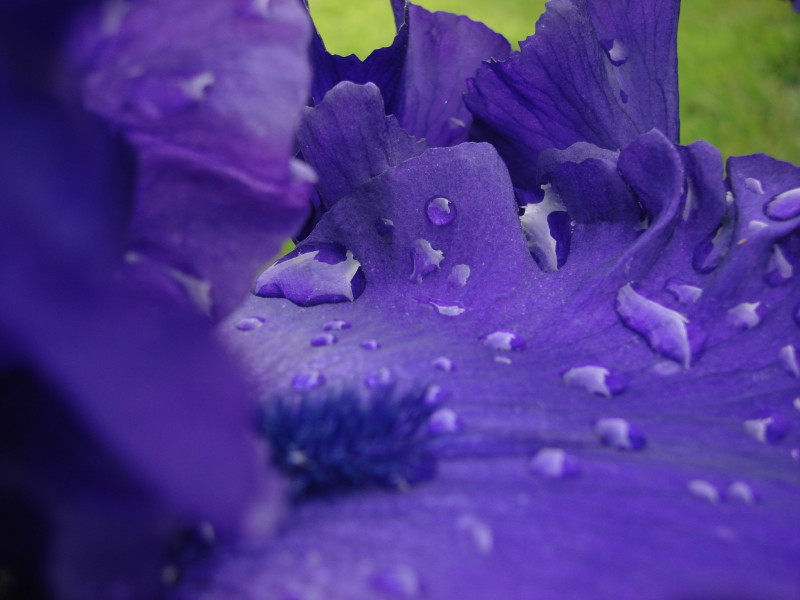This highly detailed, close-up image captures the intricate beauty of a flower, with its deep purple petals prominently magnified. The petals, adorned with glistening water droplets of various sizes, suggest the flower was recently watered or after a rain. The photograph features stunning clarity, highlighting the fine black lines that run across the purple petals. In the center of the flower, we can see a blue, fluffy-looking part, possibly the stigma, with exceptional detail. However, the left side and foreground of the image appear blurry, adding a sense of depth to the photograph. The bright green leaves and grasses in the background create a vibrant contrast, emphasizing the flower's lush color and vitality. This image was taken outdoors during the daytime, showcasing the flower in its full, healthy glory.